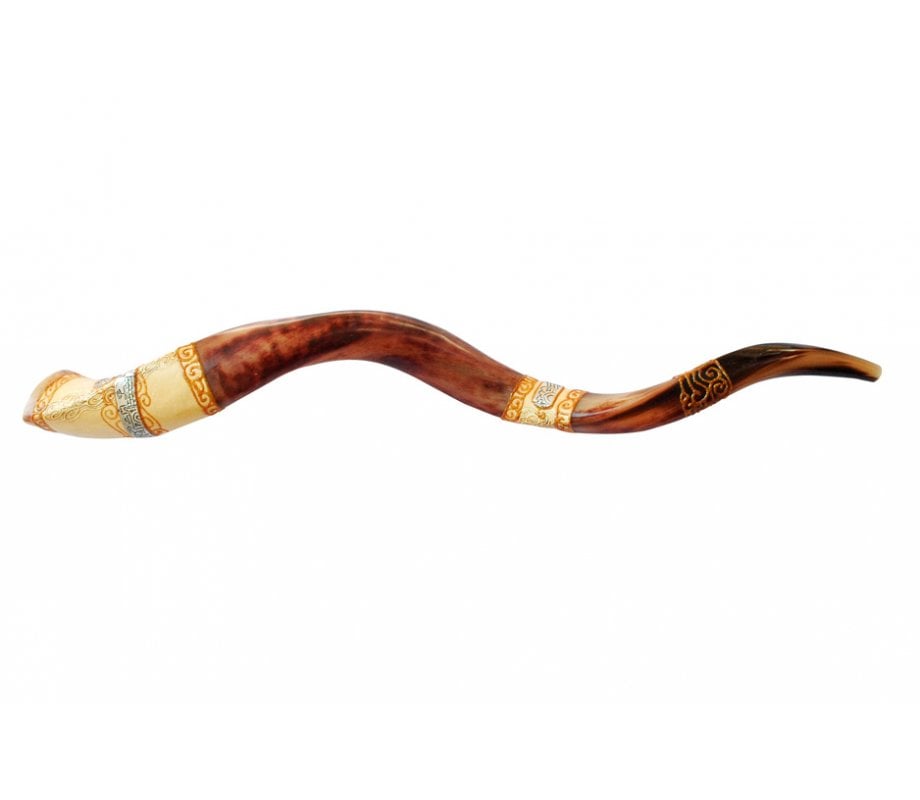The image depicts a ceremonial staff-like ornament, possibly crafted from wood, bone, ivory, or an animal's horn. The object is displayed horizontally across a white background, curling and twisting like a snake. It has an uneven, highly polished surface, predominantly a rich cherry wood color with speckled brown and black hues. The staff features intricate carvings and embellishments, including two distinctive yellow-orange bands—a smaller one at the left tip and a larger one three-quarters of the way along the staff. These bands appear to be made of either paper or metal, contributing to the object's elaborate design. Despite its smooth, glossy finish and intricate details, its exact purpose and size remain unclear.